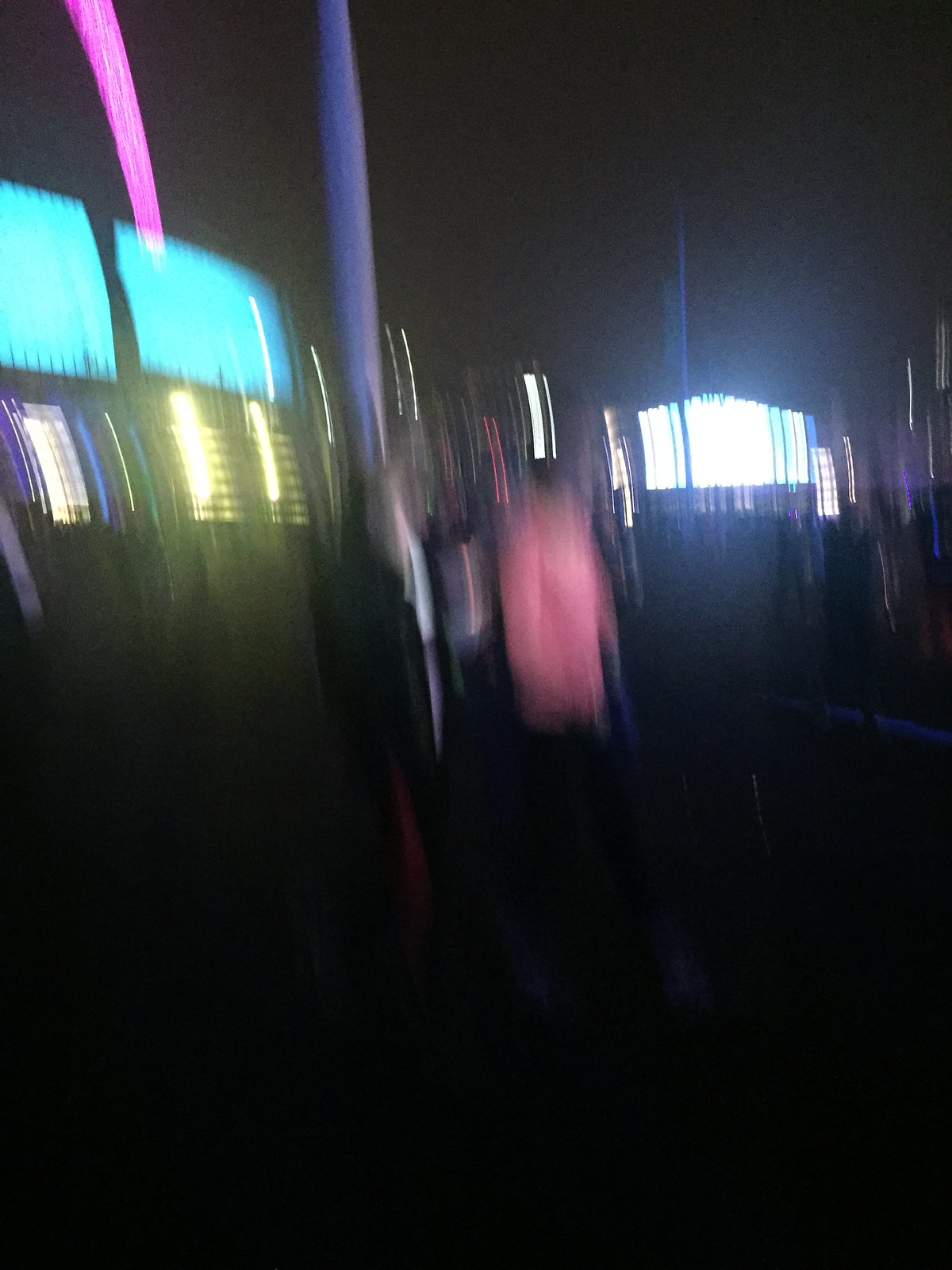The image depicts a slightly blurred and somewhat distorted scene, possibly due to camera shake or an accidental bump. Despite the blurriness, it appears to show a lively and colorful environment, hinting at a public place filled with vibrant lights. On the left side of the image, there are illuminated machines, which suggest the setting might be a casino or an arcade. The distinctive square shapes and bright lights typical of gaming machines reinforce this impression. In the foreground, two people are visible, one clad in a black jacket and the other in a light pink shirt. The overall atmosphere evokes the bustling vibe of a gaming or entertainment area, bustling with activity and excitement.